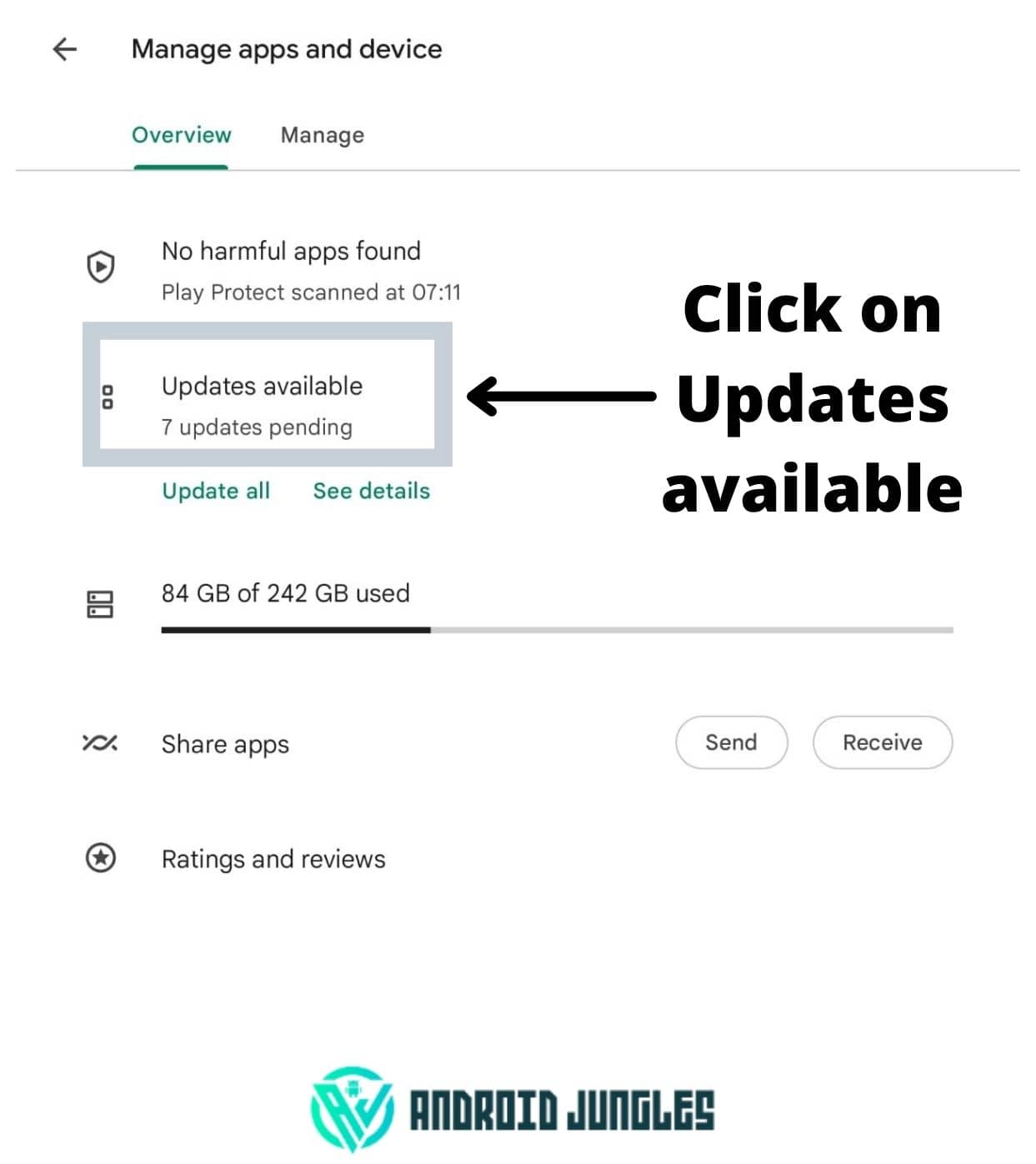The image displays an interface titled "Manage Apps & Device" at the top in black text, accompanied by a leftward-pointing arrow. The section is divided into two tabs: "Overview," highlighted and underlined in green, and "Manage," in black. It indicates that no harmful apps were found, with Play Protect having scanned at 7:11. A shield icon with a right-pointing triangle is adjacent to this information.

Below, a prominently bordered gray box states "Updates available, 7 updates pending," with a large black arrow pointing towards it and text instructing to "Click on updates available." 

Further down, storage usage is detailed as "84 GB of 242 GB used," illustrated by a black bar filled about a quarter of the way. The options "Share apps," "Send," and "Receive" are highlighted in gray circles. 

The section labeled "Ratings and reviews" includes a black star within a black circle to the left of the text, with the mention of "Android Jungles" in dark green beneath it. An adjacent teal-colored circle enclosing a downward-pointing triangle completes the visual elements on this part of the interface.